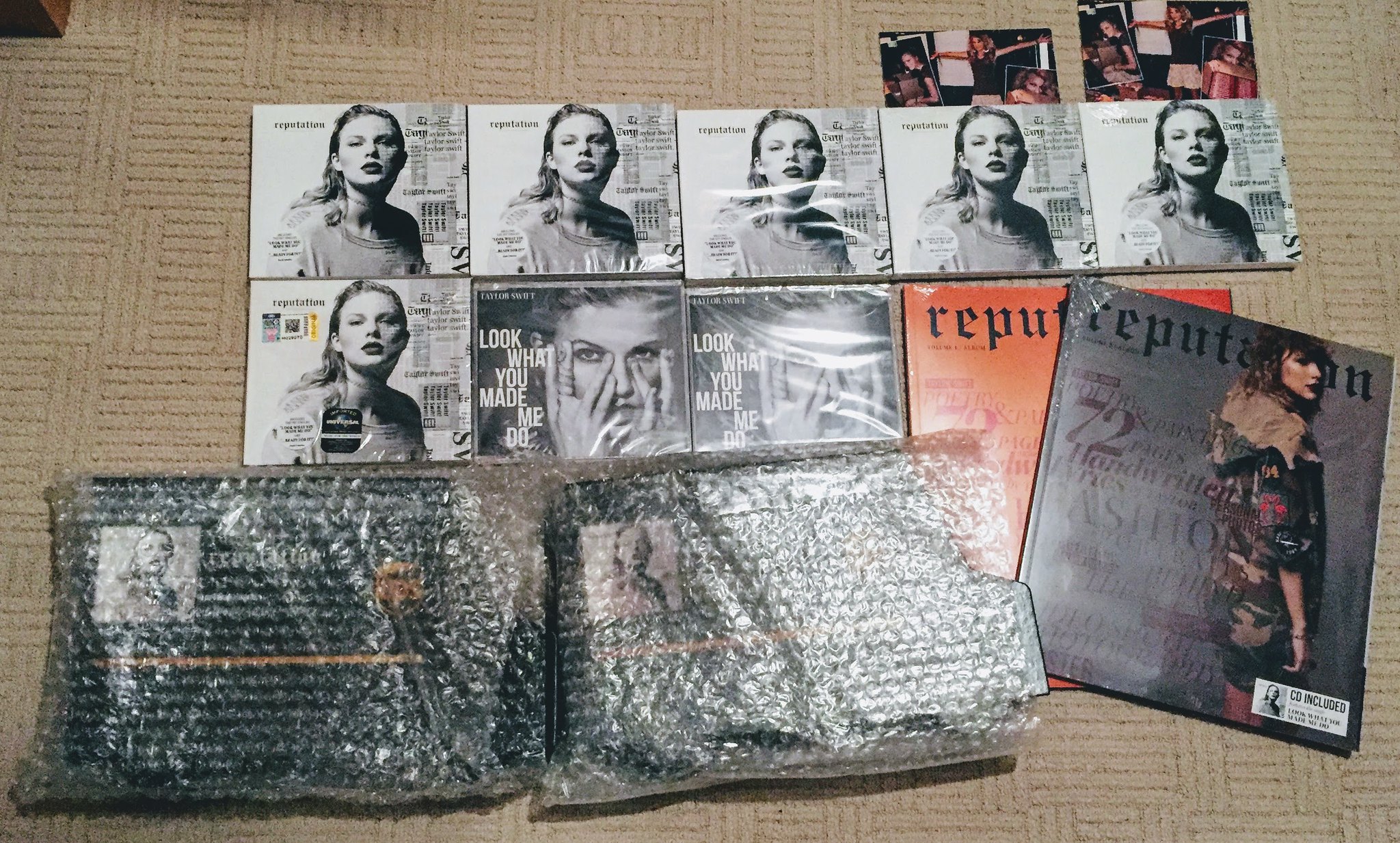This photograph showcases a meticulously arranged collection of Taylor Swift memorabilia on a beige, flat carpet that mimics the look of parquet flooring. The collection includes eight CD covers prominently featuring the "Reputation" album artwork, characterized by Taylor Swift with slicked-back hair, a choker, and an off-the-shoulder t-shirt, alongside newspaper-like columns on the right. Accompanying the CDs are two magazines—one displaying Taylor Swift in camouflage and gray hues atop an orange background—further highlighting the "Reputation" era. Additionally, there are two boxy items encased in bubble wrap, through which Taylor Swift's image is visible. In the upper right corner, two photographs depict moments likely featuring Taylor Swift and fans. A table or chair leg peeks in from the top left, hinting at the room's setting. This carefully curated collection appears to be a personal showcase of cherished Taylor Swift memorabilia, some items still preserved in plastic wrap for protection.